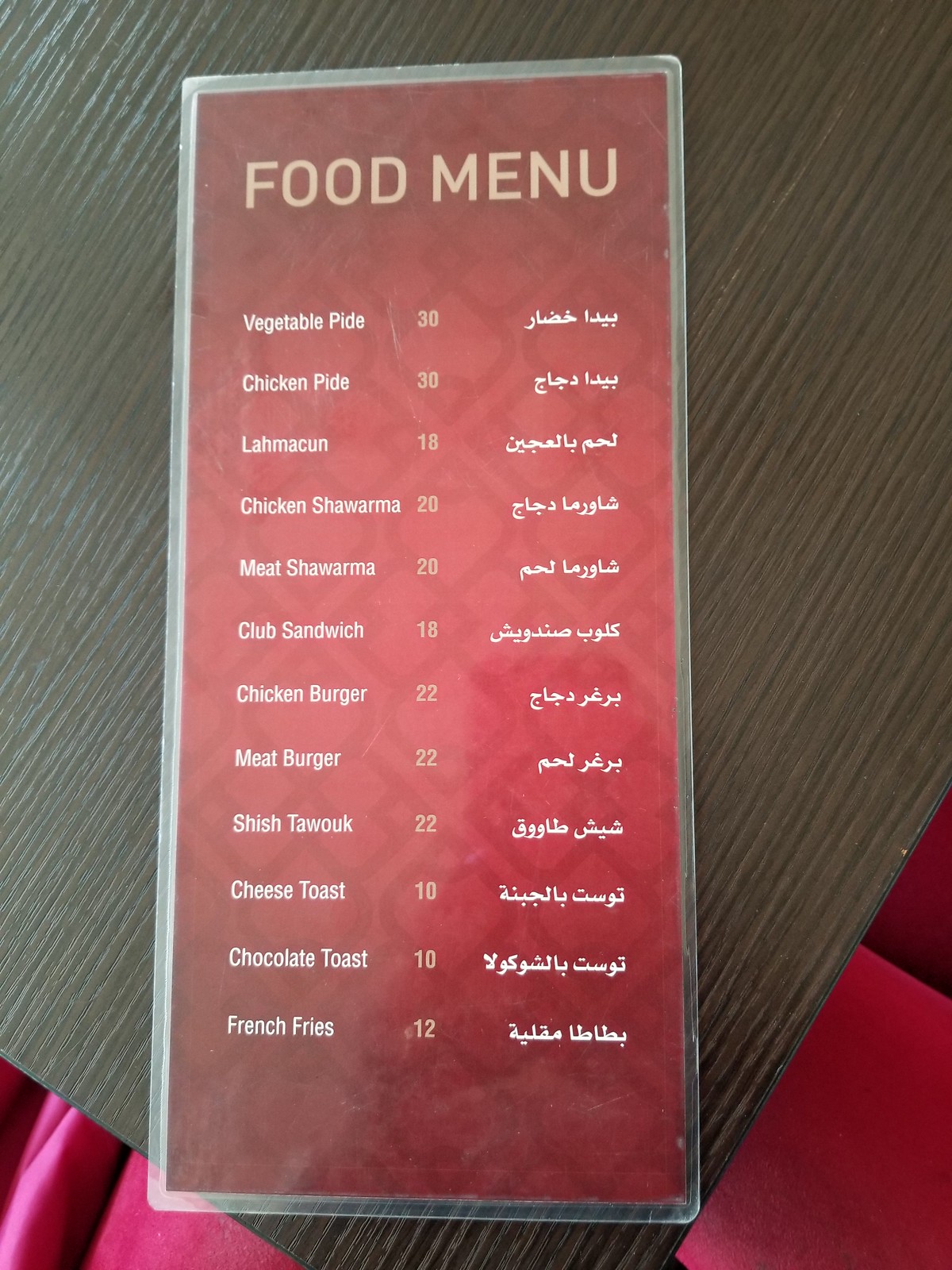In this photograph, the focal point is a tall, laminated food menu set against a dark red background with "Food Menu" written in yellowish lettering at the top. The menu, which appears to be placed on top of a dining table with a distinctive, long, grainy, fibrous texture, lists various food items. 

From the top left, the menu features:
- Vegetable Pied: $30
- Chicken Pied: $30
- Lamb Coon: $18
- Chicken Shawarma: $20
- Meat Shawarma: $20
- Club Sandwich: $18
- Chicken Burger: $22
- Meat Burger: $22
- Schistwok: $22
- Cheese Toast: $10
- Chocolate Toast: $10
- French Fries: $12

The menu appears bilingual with English on the left side and Arabic on the right. Additionally, a light, lacy pink fabric, possibly a decorative table lining, is visible in the bottom left and right corners, adding a delicate touch to the rustic table setting. The detailed presentation of the menu and the textured surface of the table highlight the variety of items available for ordering.